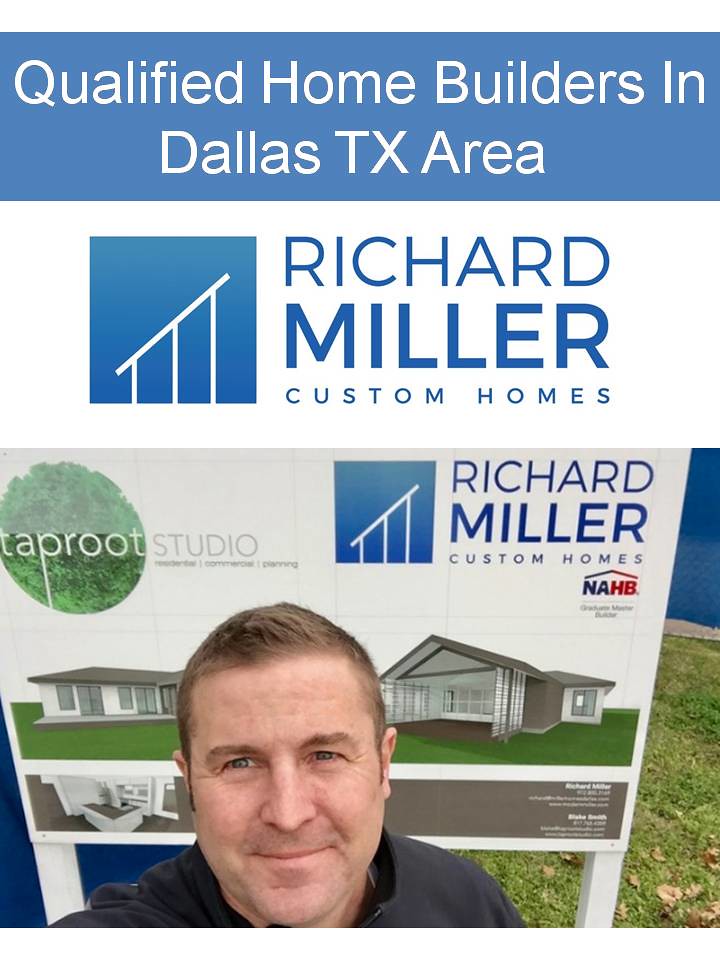This advertisement for Richard Miller Custom Homes showcases their brand in the Dallas, Texas area. The top part of the image features a light blue background with white text stating "Texas Qualified Home Builders in Dallas, Texas Area," followed by "Richard Miller Custom Homes" in blue text against a white backdrop. To the left, there's a blue box logo displaying a white stair railing. 

In the lower part of the image, a man, likely Richard Miller, is looking directly at the camera as if taking a selfie. He has short brown hair and is wearing a black shirt. This image of him is set against a yard advertisement sign that prominently displays the words "Taproot Studio" with a green circle behind it on the left side. To the right, the Richard Miller Custom Homes logo reappears, accompanied by a computer-generated rendering of his custom homes. The sign is mounted on two white wooden stakes, with green grass visible behind it.